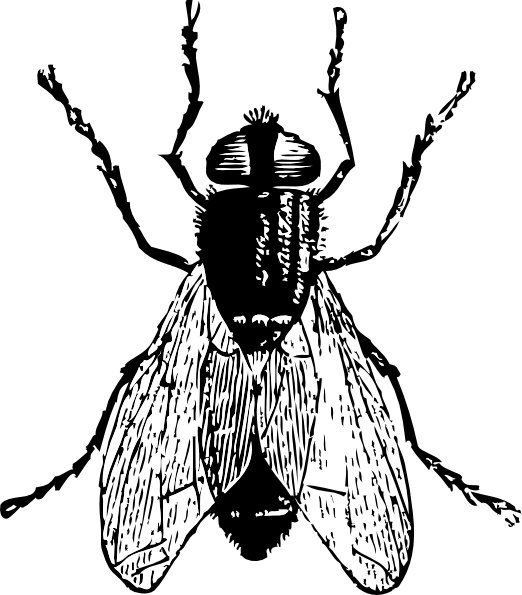This image is a black ink silhouette sketch of a housefly set against a white background. The sketch, while more of an artistic rendering than a scientific one, presents a top-down view of the fly with intricate, exaggerated details. The fly features a dark, hairy body with a distinct, slightly feathered and pointy rear end. Its head is defined by large, simply illustrated black eyes with horizontal lines. From the body, three pairs of legs extend: the front pair pointing forward, the middle pair angling towards the upper corners, and the rear pair towards the lower corners, each ending in detailed pinchers. The wings are stark white and drawn in a minimalist, artistic style, adding to the overall simplicity of the sketch.